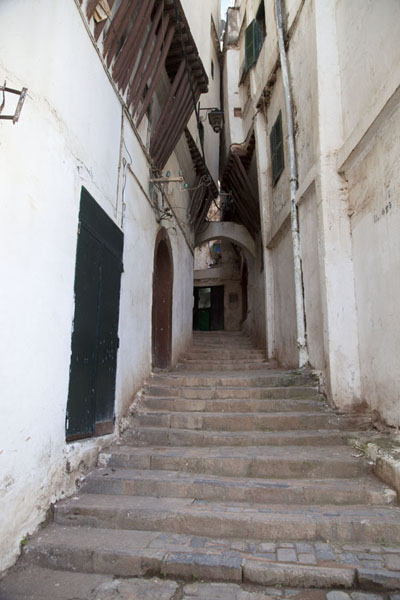This vertical photograph captures a picturesque European alleyway, possibly in Spain or Italy, framed between two ancient stone buildings. The cobblestone steps ascend through the narrow passage, guiding the eye uphill. On the left, an old white building boasts a green door and green-shuttered windows on the second and third floors. The second floor also features a porch-like structure with wooden slats for support. On the right, a similarly-aged building displays a weathered black door and a prominent pipe climbing up its wall. Both buildings exhibit a series of balconies and a brown arched doorway at one point, adding to their charm. The close proximity of the buildings, with tops almost touching, creates an intimate and slightly enclosed atmosphere. This alleyway, with its unique architectural elements and narrow passage, invites visitors for a leisurely stroll through its historic embrace.